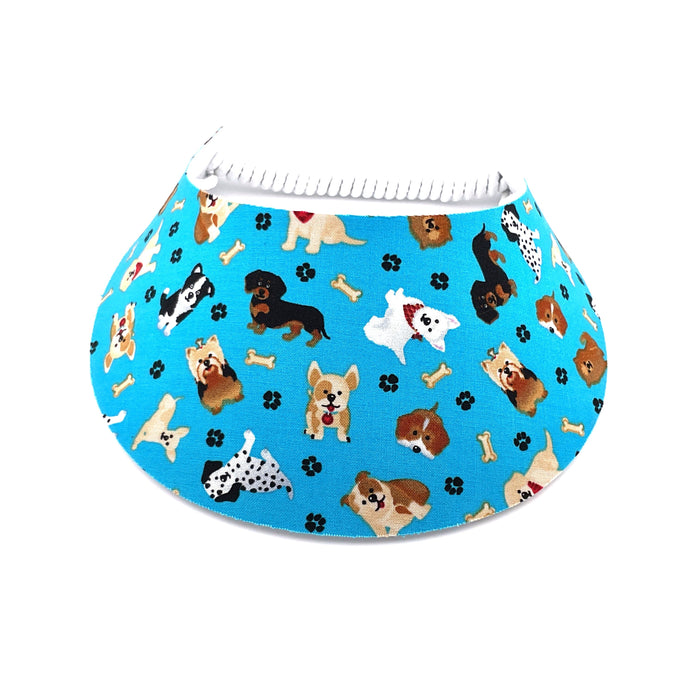This is a color photograph of a blue sun visor, designed for online shopping display. The visor features a playful pattern of cartoon dogs, dog bones, and black paw prints scattered across the light blue background. Various dog breeds are depicted, including Dalmatians, brown and white bulldogs, and dachshunds, all illustrated in a minimalistic yet charming style. The visor has a curved brim that ends on both sides and is held in place by a white elastic strap visible at the back. The photograph is set against a plain white background emphasizing the details of the visor.